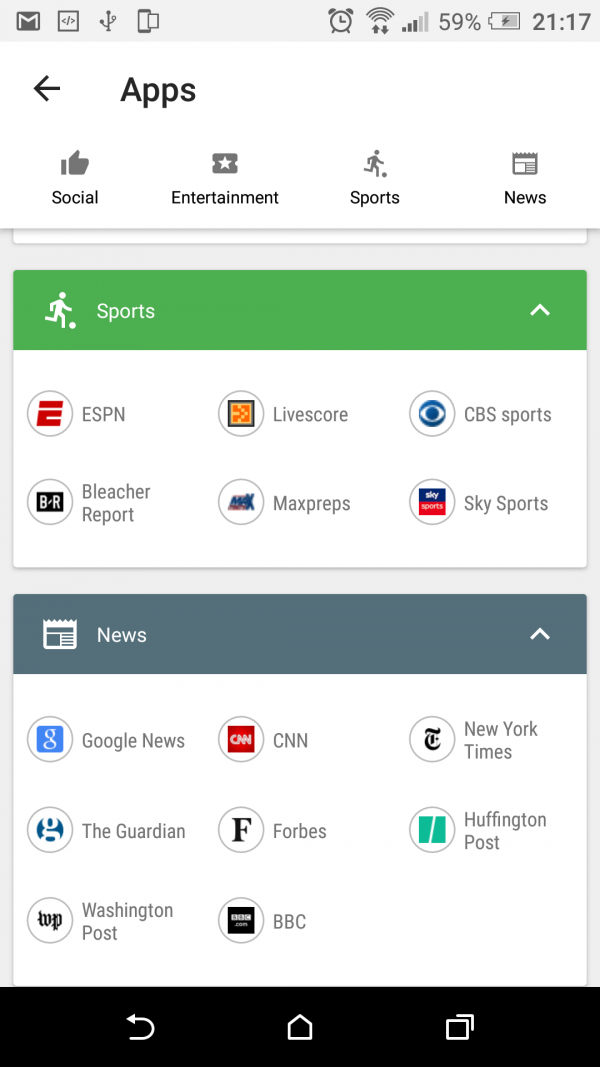This screenshot displays the interface of a mobile phone, detailed from top to bottom. 

At the top of the screen, there is a prominent Google Mail icon resembling an envelope with the letter "M." Adjacent to this is a box containing a less-than sign, a forward slash, and a greater-than sign, which typically represents HTML tags. Next to this box, there is an icon that looks like a coat rack: a long pole with lines extending from the bottom, middle, and top, each with circles at their ends. Following this, there is an icon depicting a phone, and another square beside it. 

The status bar indicates that an alarm is set, Wi-Fi is enabled, the signal strength is at three bars, the battery is at 59%, and the current time is 21:17 (9:17 PM). Below this, a black arrow pointing to the left is labeled "Apps."

Underneath the "Apps" label, there are four monochromatic icons categorized as follows:
1. A thumbs-up icon represents "Social."
2. A ticket with a star inside represents "Entertainment."
3. A stick figure playing soccer represents "Sports."
4. A newspaper icon represents "News."

Specifically, the "Sports" category is highlighted in white text on a green background with a white arrow pointing up, indicating that the menu can be hidden. The icons for sports apps within this category, all encased in white circles, include:
- ESPN (E inside a white circle)
- Bleacher Report (BR in a white inside a black rectangle)
- LiveScore (black square paired with an orange square featuring a yellow dotted right arrow)
- CBS Sports (CBS logo resembling an eyeball)
- MaxPreps (word "MAX" with a prominent blue "X")
- Sky Sports (blue rectangle with "Sky" in white text and a connected red rectangle with "Sports" in white text).

Following this section, the "News" category is displayed with a white arrow indicating it can be collapsed. The "News" label is in white text on a grayish-blue background, with icons including:
- Google (white "G" in a blue square)
- CNN (red square with white "CNN")
- The New York Times (stylized "T")
- The Guardian (white "G" in a blue circle)
- Forbes (black "F")
- Huffington Post (aqua page with a diagonal slice)
- Washington Post (white "WP" in black text)
- BBC (black with white "BBC" in black text within white boxes).

At the bottom of the screenshot, there's a black rectangular navigation bar with three icons:
- A "U" turned on its side with an arrow pointing left (possibly the 'Back' button)
- A house icon (likely the 'Home' button)
- A square with the top-right corner of another square behind it (probably the 'Overview' or 'Recent Apps' button).